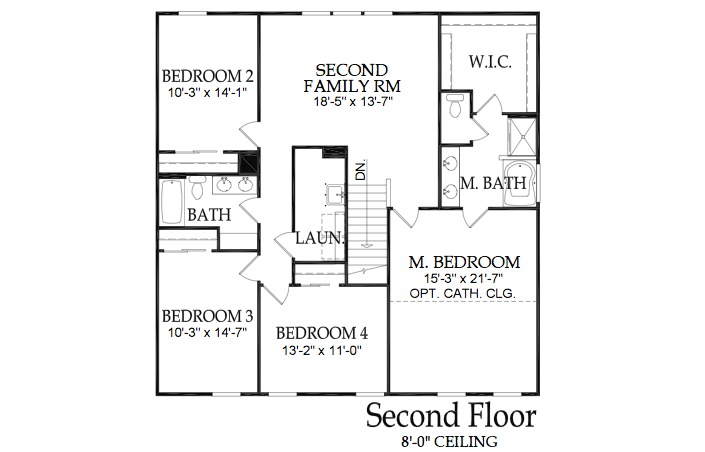Diagram Depicting Second Floor Plan: 

The diagram illustrates a comprehensive layout of a second floor plan, encapsulated within a vertically oriented rectangle. In the top-left corner, the plan indicates "Bedroom 2." Moving towards the center, a "Second Family Room" is prominently featured. Adjacent to this family room, labeled "W-I-C," is a walk-in closet with a connecting door leading to the "M. Bath," the master bathroom.

Prominently positioned in the central area is a room labeled "L-A-U-N," which stands for the laundry room, positioned alongside a staircase.

On the left side, another bathroom is depicted. Directly beneath this bathroom is "Bedroom 3," with "Bedroom 4" situated adjacent to it. Completing this section, in the bottom-right corner of the diagram, lies a spacious master bedroom labeled "Master Bedroom."

The bottom of the diagram explicitly notes "Second Floor," alongside the specification, "8'0" Ceiling," indicating the height of the ceiling. Several spaces throughout the plan are marked for windows, effectively indicating their placement in each of the rooms.